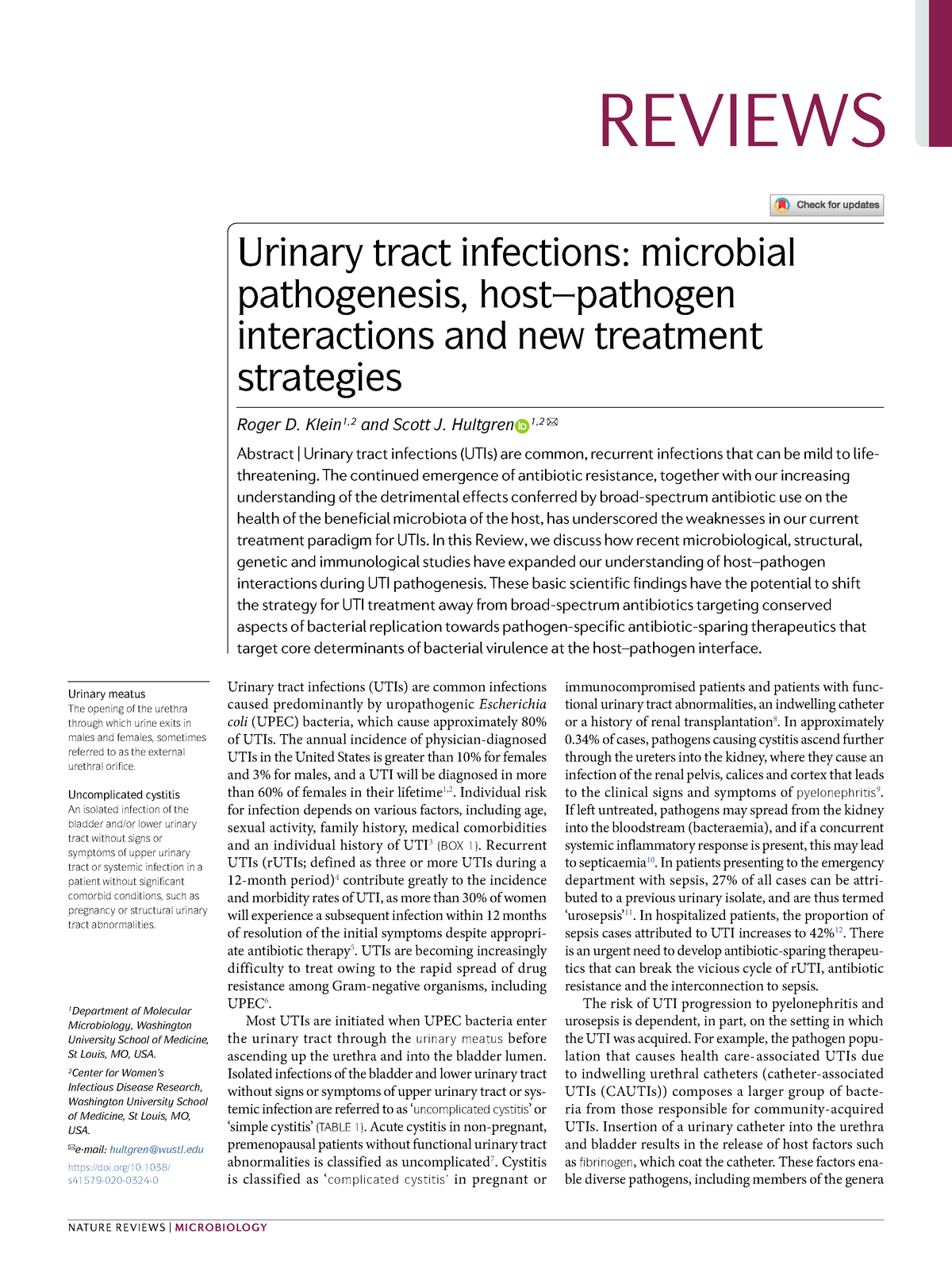"Detailed illustration showcasing the microbial pathogenesis of urinary tract infections (UTIs) and the complex host-pathogen interactions involved. The image highlights emerging treatment strategies to combat these infections. An article below delves into the intricacies of these topics, although the text is too small to read clearly."